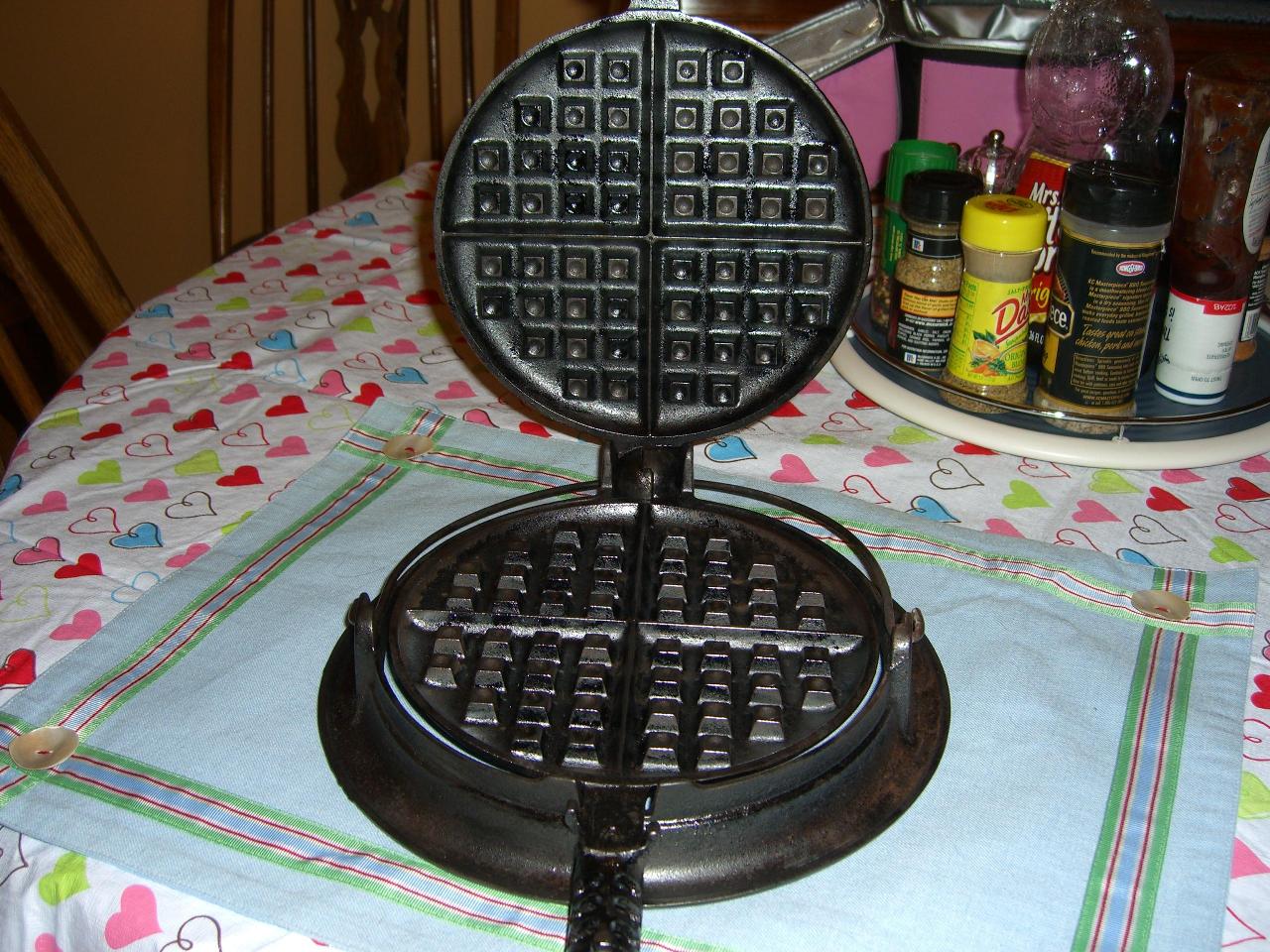In this horizontally laid, color photo, we see a close-up of an old, black, and heavily used circular waffle maker, open to reveal its four pie-chart-like sections. The rustic waffle iron, showing signs of significant wear and blackened from many uses, rests prominently at the center of a table. The table is covered in a white tablecloth adorned with colorful hearts—red, pink, blue, and white—and has a blue placemat with a green ribbon border beneath the waffle maker. Adjacent to the old appliance, towards the back, is a loaded lazy Susan displaying various spices and condiments, including brands like Mrs. Dash, McCormick, and a bottle of Mrs. Butterworth's syrup. Additionally, chairs are scattered around the table, emphasizing the homely and warm kitchen setting.